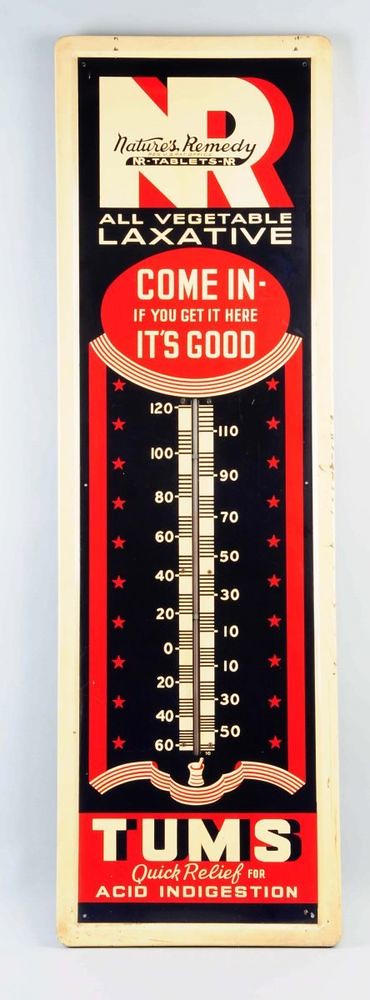This vintage photograph captures an antique thermometer that serves as an advertising piece for Tums, the well-known remedy for acid indigestion. This vertical, rectangular thermometer is crafted from metal and has an authentically aged appearance. The outer border is a gentle cream color, which frames the piece beautifully.

At the very top, the logo reads "N.R.," which stands for Nature's Remedy, accompanied by the text "N.R. Tablets" beneath it, all set against a rich black background. Below the logo, in smaller lettering, is the slogan, "All Vegetable Laxative." A prominent red circle on the piece contains the inviting text, "Come in. If you get it here, it's good."

Central to the design is the thermometer itself, running down the lower center of the piece. The scale is marked by red lines and punctuated by red stars along the edges, giving it a distinct and eye-catching appearance.

At the bottom, a horizontal text bar carries the bold, reassuring words, "Tums, Quick Relief for Acid Indigestion," making this not just a functional item but also a historic artifact of medical advertising.